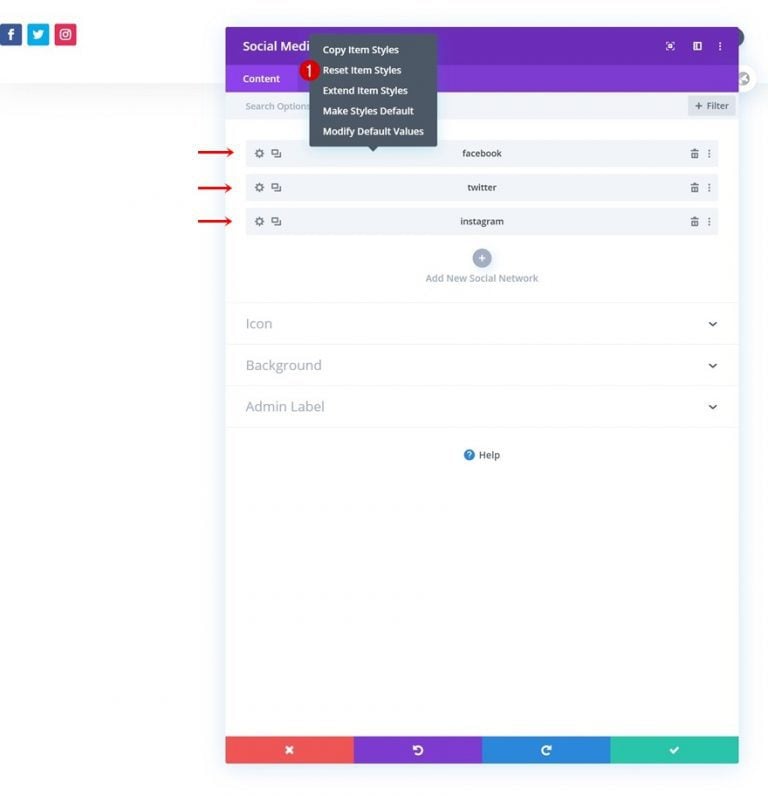**Detailed Descriptive Caption:**

This image is a smartphone screenshot displaying a user interface with various social media platform logos and a well-structured pop-up menu. At the top of the screen, prominently visible, are the logos of Facebook, Twitter, and Instagram. The page is framed with a purple border, with a lighter shade of purple following beneath it. Within this lighter purple section, partially obscured by a black drop-down box, the text "social media" is visible.

The drop-down box contains a vertical list of options, which read: "Copy item styles," "Reset item styles," "Extend item styles" (repeated twice), "Make styles default," and "Modify default values."

To the left, in the lighter purple area, there's a heading labeled "Content," immediately followed by a search options box. On the far right, a filter button featuring a plus symbol can be seen.

The page also has several arrows pointing to three distinct sections, each equipped with a settings wheel and a double-screen icon. Centrally aligned, the names of the social media platforms—Facebook, Twitter, and Instagram—are listed vertically. Next to each platform name, on the right side, are trash can icons, followed by three vertical dots indicative of additional options.

At the bottom portion of the screen, a plus button labeled "Add new social network" invites users to integrate more platforms. Further below, there are three entries, labeled respectively as "Icon," "Background," and "Admin Label," each accompanied by a drop-down arrow on its right side. Accompanying these is a question mark icon with "Help" written beside it.

Finally, a colorful set of tabs at the very bottom displays four buttons: a red tab with an 'X' signifying a crossout, a purple tab with a refresh icon, a blue refresh button, and a green tab with a check mark, completing the vibrant layout and user interface options.